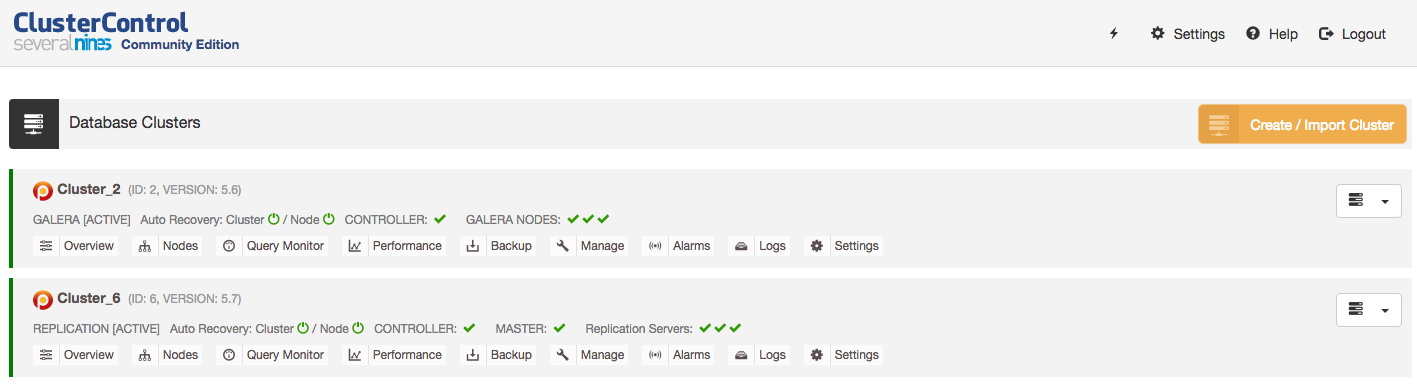In the top left corner of the image, the heading "Cluster Control" is prominently displayed, with "Several Nines Community Edition" written below it. In the top right corner, there are options for "Logout," "Help," and "Settings." Adjacent to these labels are corresponding icons: a door icon next to "Logout," a circle with a question mark next to "Help," and a gear icon next to "Settings." A lightning bolt icon is situated just left of the gear icon.

At the center-left of the image, the phrase "Database Clusters" appears alongside a small black square containing a computer icon. On the far right of these words, an orange button labeled "Create / Import Cluster" stands out.

In the bottom left area, there are two sections. The first section is labeled "Cluster 2 ID 2 version 5.5." Under this label, several categories are listed: "Overview," "Nodes," "Query Monitor," "Performance," "Backup," "Manager," "Log," and "Settings." Below this is another section labeled "Cluster 6 ID 6 version 5.7," which includes the same categories as the section above.